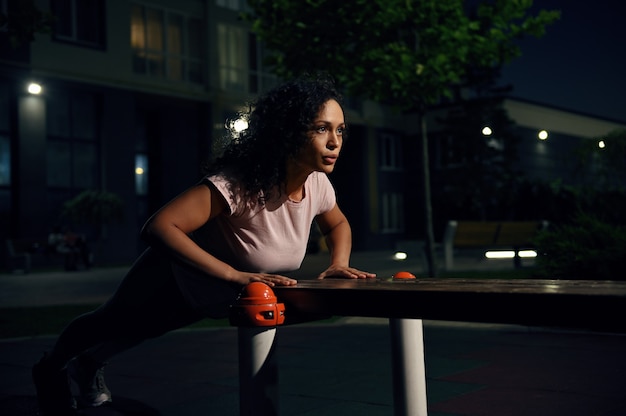In this nighttime photograph set in an urban environment, a determined-looking black woman with long, wavy dark hair is captured in mid-exercise. She appears to be stretching or performing a push-up against a piece of exercise equipment featuring white posts with orange caps and a broad black horizontal beam. She's wearing a pink short-sleeved shirt, leggings, and running shoes. The scene behind her includes typical residential apartment buildings illuminated by streetlights, a park bench with metal legs and orange caps, and a small tree along the sidewalk. The woman stands slightly to the left of center, exhaling sharply, her palms spread outward and elbows bent as she leans into her stretch. The photograph, in landscape orientation, utilizes photographic representationalism realism to capture the urban ambiance against the darkened background.